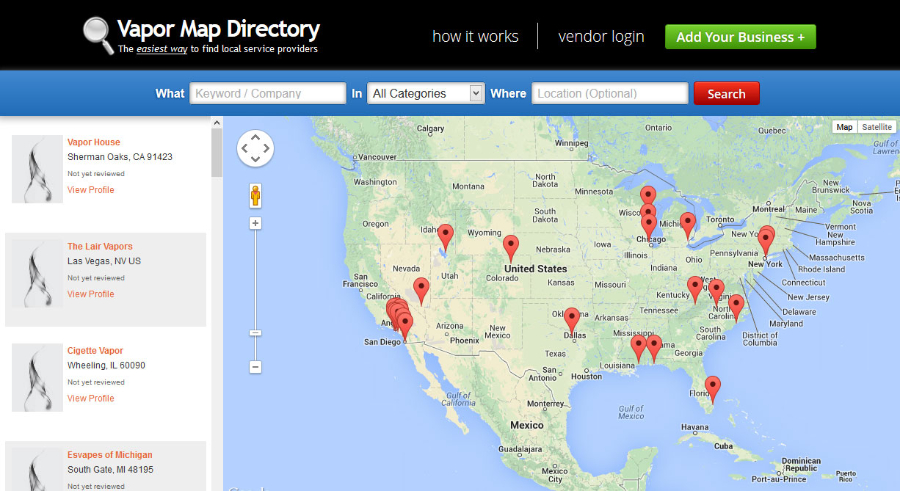Screenshot of a website featuring a large map of the United States. The top black bar displays "Left Paper Map Directory," followed by the tagline "The easiest way to find local service providers." To the right, there are links labeled "How It Works" and "Vendor Login." A green button with white text prompts users to "Add Your Business."

Beneath this header, a blue bar contains search functionalities. The "What" field includes an input box for keywords or company names, followed by a drop-down menu labeled "All Categories." The "Where" field features an optional location input box, accompanied by a red "Search" button.

On the left side, a sidebar lists various locations with accompanying images and descriptions. The main section on the right showcases a large, detailed map of the United States dotted with red pins. A plus and minus slider on the left side of the map allows users to adjust the zoom level.